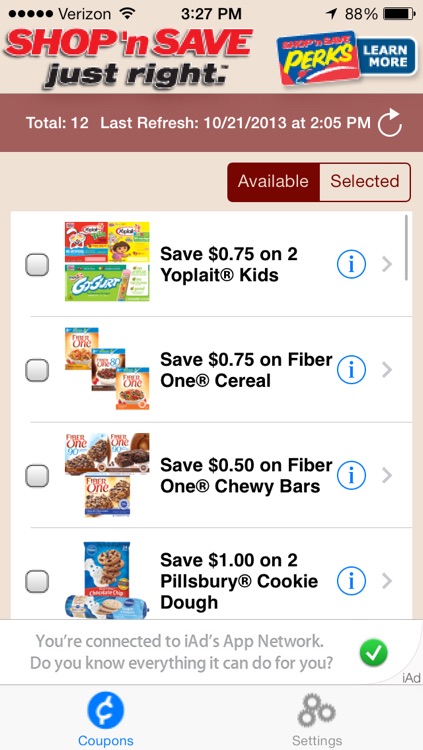**Detailed Caption:**

The screenshot features a smartphone on the Verizon network, displaying full cellular coverage and an 88% battery charge at 3:27 PM. At the top of the screen, there is a prominent banner reading "SHOP AND SAVE," with all letters in bold, capitalized text, except for the 's' and 'e' at the ends, which are lowercase. The text is red and slightly italicized, leaning to the right. Directly below, in black text that is also italicized, the phrase "Just Right:" appears.

Adjacent to this banner is a section labeled "Perks," which appears as a digital card featuring a clickable option reading "Learn More." Underneath this card, it reports a total of 12 perks, with the last refresh noted on October 21st, 2013 at 2:05 PM. An option to refresh this information is available.

The main part of the screen displays two tabs: "Available" and "Selected," with the "Available" tab currently active. Listed under this tab are various items for which coupons are available, including Yoplait yogurt, Fiber One cereal, Fiber One chewy bars, and Pillsbury cookie dough. Users can connect these coupons for their shopping needs.

A footer at the bottom of the screen shows navigation options, with "Coupons" highlighted in blue, indicating the current section. To the right of this, there is another option labeled "Settings," displayed with three small circles above it, which is not currently selected. Additionally, a notification mentions, "You are connected to iAds app network. Do you know everything it can do for you?" accompanied by a small checkmark.

This detailed view offers users a convenient way to manage and select shopping coupons directly from their smartphones.